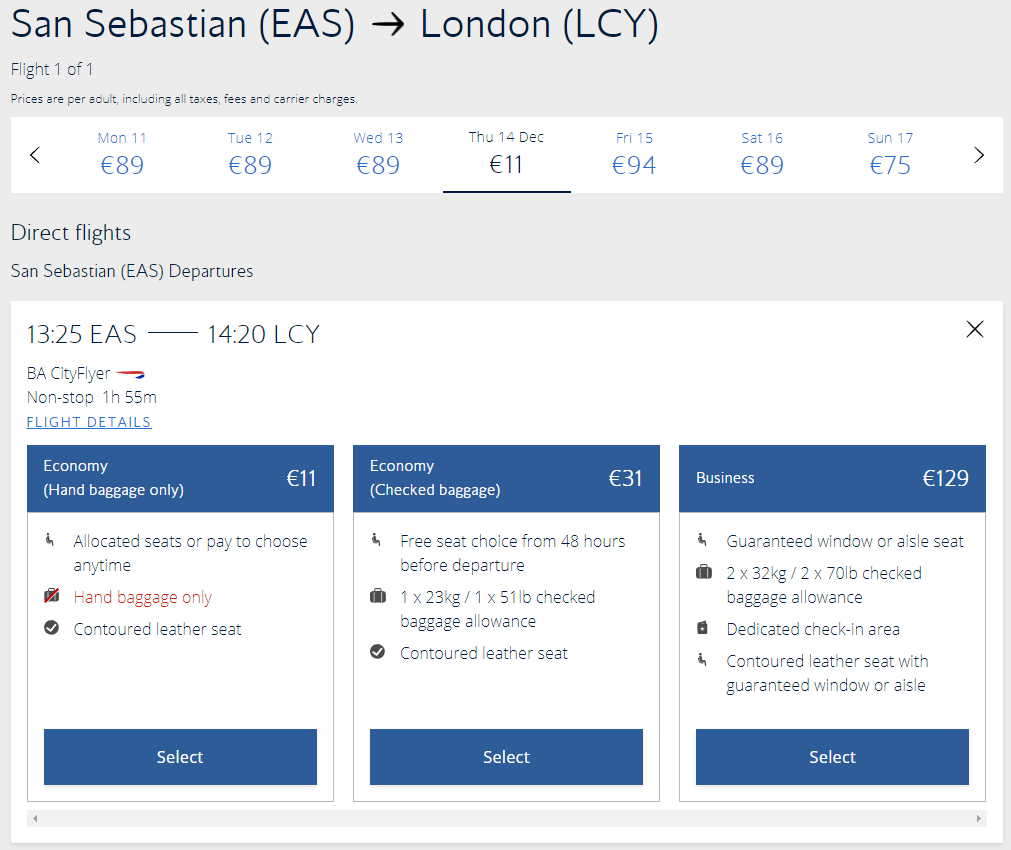**Flight Itinerary from San Sebastian to London**

This screenshot depicts a flight itinerary from San Sebastian (EAS) to London (LCY), organized within a gray interface with multiple white segments. 

At the top, the display reads "San Sebastian to London," indicating the singular flight option available. A horizontal white slider below enables selection across various dates and corresponding prices:

- **Monday, 11:** €89
- **Tuesday, 12:** €89
- **Thursday, 14:** (highlighted in black and underlined) €11

Most dates on the row are depicted in blue, except for the prominently featured Thursday, December 14th, marked in black and underscored, signaling the exceptionally low fare of €11.

Under this date selector, the text "Direct flights" appears, followed by a detailed flight schedule:
- **13:25 EAS to 14:20 LCY** 
Indicating a direct, non-stop flight of 1 hour and 55 minutes on a BAC To Flyer aircraft. There's also a hyperlink provided for additional flight details.

Beneath this flight information, three boxed options with blue headers detail different fare classes and their respective prices:
- **Economy Hand Baggage Only:** €11 (highlighted in red text for the baggage restriction)
- **Economy Checked Baggage:** €31
- **Business Class:** €129

Each option includes a blue "Select" button at the bottom. The content within each box varies based on the fare class:

- **Economy Hand Baggage Only:** Basic fare for those traveling light.
- **Economy Checked Baggage:** Includes a checked baggage allowance.
- **Business Class:** Offers numerous benefits such as a dedicated check-in area, contoured leather seating with the guarantee of a window or aisle seat, and double baggage allowance.

Overall, the screenshot provides a comprehensive overview of flight options, pricing, and amenities for travelers flying from San Sebastian to London.